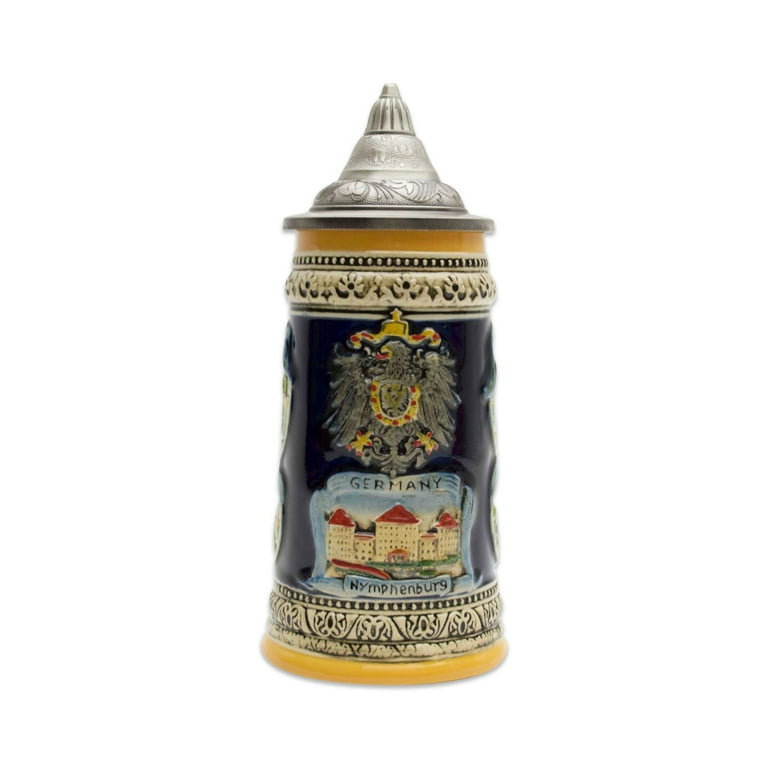The image prominently features a traditional German beer stein adorned with intricate and elegant details. The stein is primarily ceramic and boasts a smooth yellow gold base layer, followed by a patterned section of black and white. Central to the design is a vivid depiction of the Nymphenburg village, accompanied by the words "Germany" and "Nymphenburg" inscribed below it. Above the village image, the crest of Nymphenburg is prominently displayed, showcasing an eagle facing to the left and adorned with several gold markings and a gold crown with red accents. The background includes a captivating black and gray swirly pattern, adding depth to the imagery. The stein's cylindrical body also features repeating black and white layers with a series of black lines interspersed with white spots. Topping this exquisite piece is a beautifully detailed pewter lid, engraved with intricate leaf carvings, shaped in a dome to complete the traditional look. Although the handle is not visible as it faces away, the overall craftsmanship and ornamental details suggest it serves as a cherished souvenir, likely representing a memorable visit to Germany.